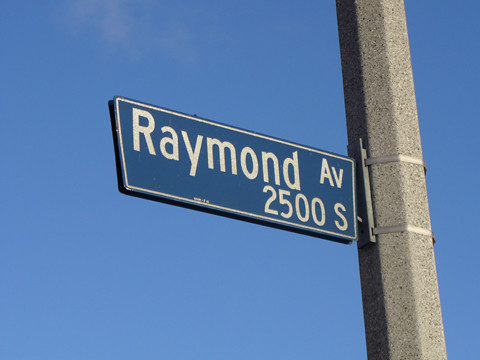In this outdoor photograph, a blue street sign reading "Raymond Avenue, 2500 South" is prominently displayed, securely fastened to a weathered concrete post with metal straps and a girder. The bright midday sun casts a clear light over the scene, highlighting the vivid blue of the sign and the slight, fluffy clouds scattered across the otherwise clear sky. The image resolution suggests it was captured with an older camera, adding a nostalgic touch to the photograph. The overall composition offers a simple yet evocative glimpse of an everyday urban setting, bathed in the crisp light of midday.